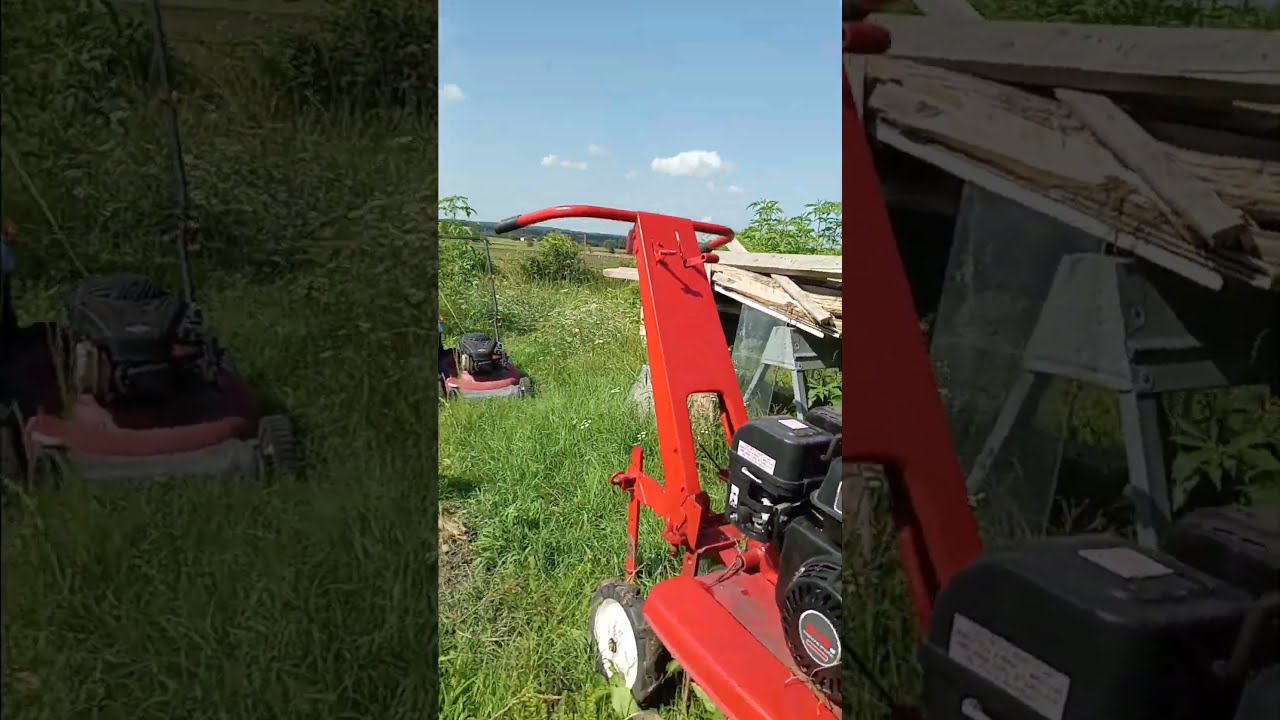The central image is set outdoors, framed by a vibrant blue sky with a few scattered clouds. The background reveals a lush, green field, surrounded by brush and small trees, with rolling hills or low mountains in the distance. The split-screen format includes close-ups to the left and right, each highlighting distinct sections of the scene.

Prominently featured is a red push lawnmower situated towards the left of the image. This lawnmower is clearly detailed and is one of the focal points. To the right of the lawnmower, partially hidden, lies another piece of red equipment. This appears to be a wood chipper or a tiller, identifiable by a small black engine and handles that emerge from its rear. Adjacent to this, there is a silver stand holding wood, resembling a pommel horse structure. The vivid colors in the image include reds from the equipment, blacks from the machinery elements, and the overwhelming greens of the tall, healthy grass. There are no people or text within the image, which overall conveys a serene outdoor farm setting.